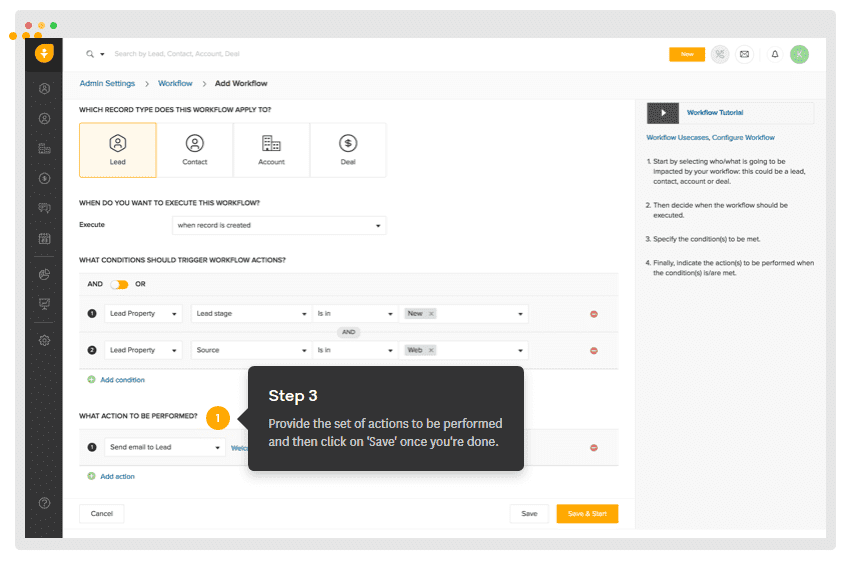Detailed Caption: 

The user interface displayed is set against a white background with a gray border at the top, featuring an array of multicolored circular icons: pink, yellow, green, and three shades of orange. Below, the screen has a search bar labeled 'Search by league, contact, account, or deal'. To the right, an orange banner with white text reads 'Now', accompanied by four circular icons. Among these icons is a bell, a green circle with an indistinguishable detail, a black envelope, and a gray-shaded icon resembling a small plant. Further to the right, options titled 'Admin Settings' and 'Workflow' are written in blue, with 'Add Workflow' in black next to them.

Below these elements, sections labeled 'Lead', 'Contact', 'Account', and 'Deal' are displayed with respective icons: a person in a hexagon for 'Lead', a person in a simple circle for 'Contact', two buildings for 'Account', and a dollar sign in a circle for 'Deal'. The 'Lead' section is highlighted in orange, while the others are shaded in gray.

Underneath, a prompt asks 'When do you want to execute this workflow?', followed by a selectable 'Execute' option and a banner suggesting 'When record is created'. Another section asks 'What conditions should trigger workflow actions?', which includes toggle options 'And' and 'Or' in orange and white. Subsequent conditions are listed: 'Lead property' with 'Lead stage' set to 'New', and 'Lead property source' set to 'Web', each in their own banner with a black arrow. An option to 'Add condition' is available in blue with a green circle plus sign.

For actions, an orange circle with a white number one indicates 'Send email to lead'. Additional actions can be added via a blue 'Add action' button. A 'Cancel' button is outlined in gray with black text. A black banner labeled 'Step 3' in white partially obscures content below it and instructs users to finalize actions and save.

At the bottom, two buttons for saving are available: a white 'Save' button and an orange 'Save and Start' button. On the far right, a 'Workflow tutorial' is presented in blue, with explanatory sections: 'Workflow', 'Use cases', and 'Configure workflow', followed by a list of four items in black.